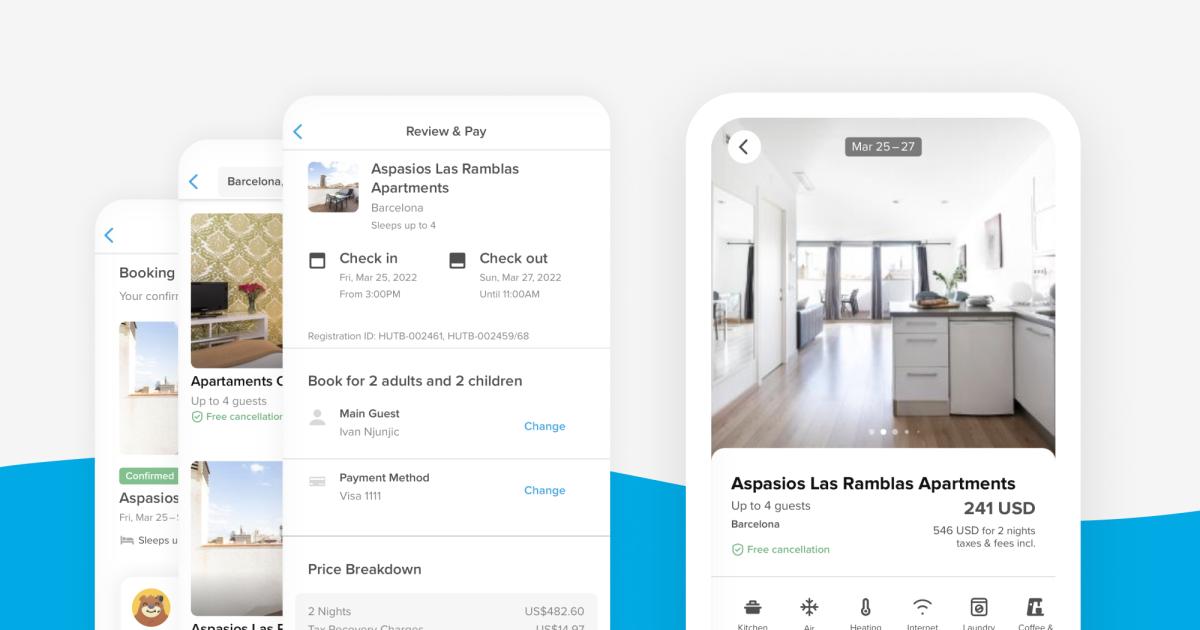The image depicts a series of three cascading mobile phone screens, likely iPhones, identifiable by the blue arrows at the top left corner of each screen. The foremost screen displays a booking interface with the header “Review & Pay” in bold black text.

Below the header, a thin light-gray divider separates the section from the main content. The image beneath this divider showcases a scene of the sky with a building or chimney visible on the right side. Below the image, bold black text reads “ASPASIOS LAS RAMBLAS Apartments,” with smaller gray text underneath stating its location, “Barcelona,” followed by “Sleeps up to 4.”

Continuing downward, the interface displays two calendar icons in dark gray. The one on the left, labeled “Check-in,” includes small light gray text beneath it reading “FRI, MAR 25, 2022” and “From 3:00 PM.” The calendar on the right is partially obscured, with its label “Check-out” showing, and small light gray text beneath stating “SUN, MAR 27, 2022” and “Until 11:00 AM.”

At the bottom of this section, there is gray text displaying the registration ID: “HUTB-002461, HUTB-002459/68.” Further below, black text clarifies the booking details: “Book for 2 adults and 2 children.”